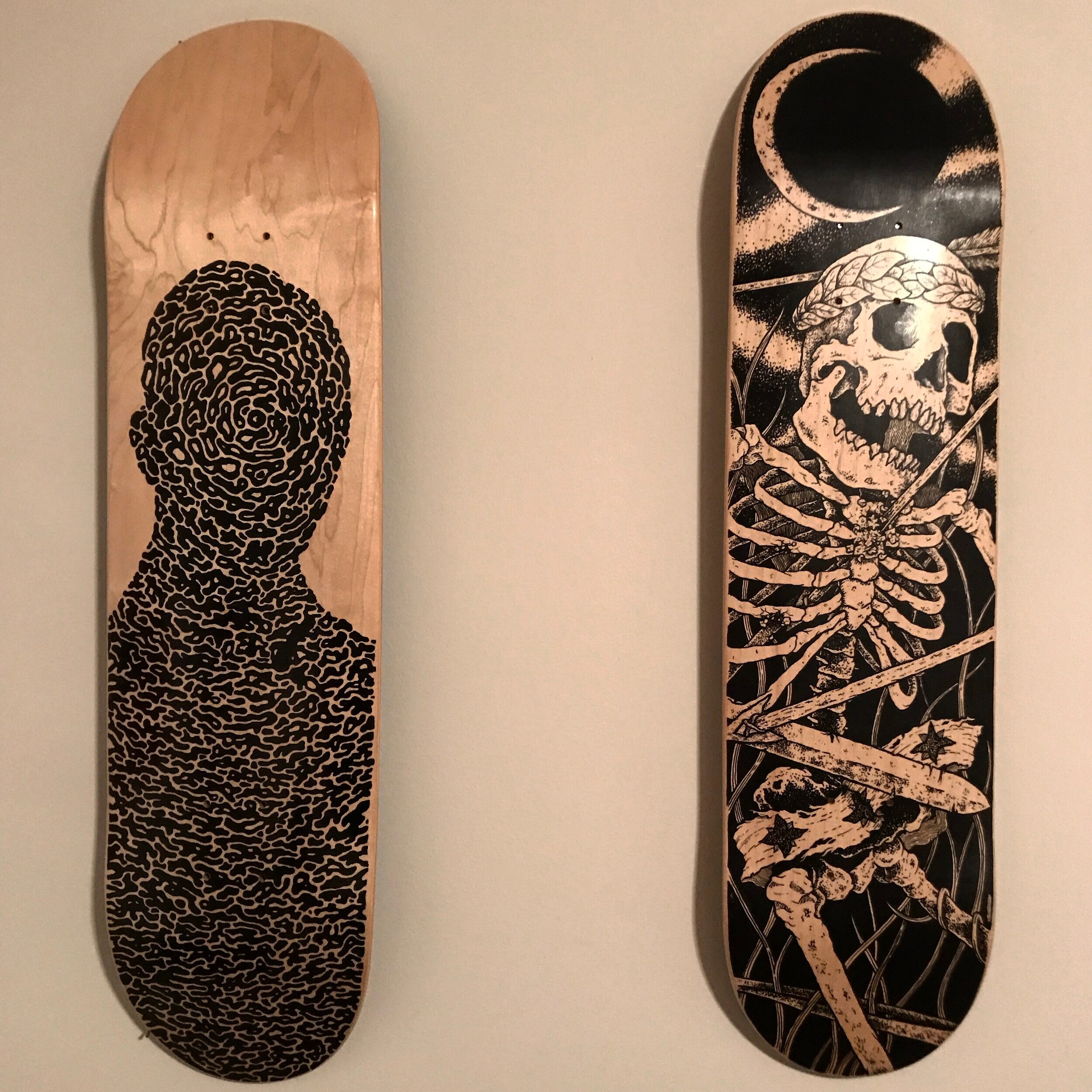This photograph captures two identical-sized skateboards, both stripped of their wheels, screws, and any labels. They are placed on a tan-colored surface, possibly a piece of paper or a floor, with slight shadows visible behind them. 

The skateboard on the left features artwork of a human figure. The design is predominantly black, with the head and chest depicted as a series of squiggly, spiral shapes, giving an abstract representation of the human form.

The skateboard on the right has a more intricate design, illustrating a skeleton adorned with symbolic elements. The skull wears a wreath-like headband reminiscent of ancient Greek crowns, and the bony figure is holding a sword. Its ribcage and hip bones are encircled by a ribbon, while a crescent moon appears above the skull. This board features a black background with additional details like gold clouds behind the moon, and the skeleton's belt has star decorations.

Both boards have visible holes where the wheels and screws would be attached, emphasizing their incomplete state.